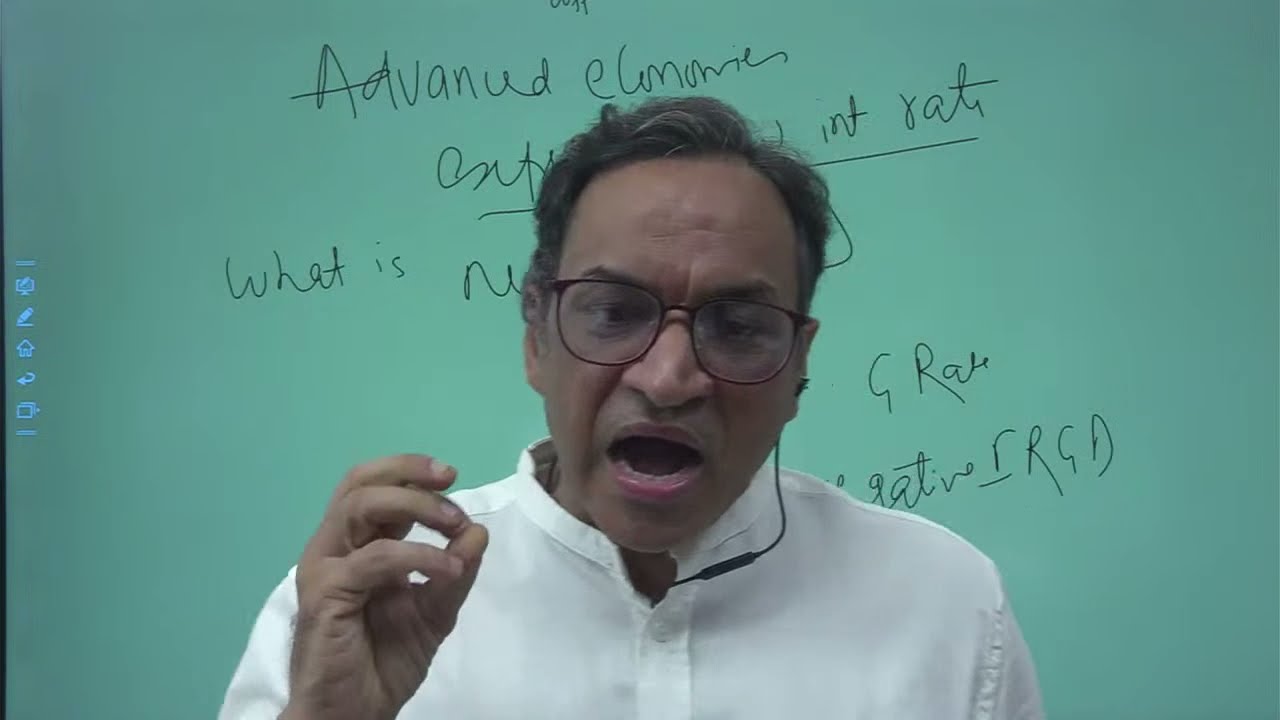This photograph is of a middle-aged man, likely of Indian or Middle Eastern descent, delivering a lecture in front of a digitally rendered bluish-green background that mimics a classroom whiteboard. The man, appearing to be in his mid-50s, wears glasses and a white dress shirt with an open collar and a pinkish sleeve. He is equipped with an earpiece microphone, indicating that he may be teaching online.

His dark, wavy hair frames a face focused intently on his lesson, his mouth open mid-speech, revealing his tongue and bottom teeth. His head tilts slightly to the right, and he gestures with his hand raised, as if emphasizing a point and making an "okay" gesture with his fingers. 

The background contains partially obscured text. Visible words include "advanced economies," "interest rates," and "what is." Some letters are partially obscured by his figure, including fragments like "I-N-T," "R-A-T-E," and "negative R-R-G-D." Additionally, small icons on the left of the background suggest it is a digital screen with home and duplicate screen buttons, highlighting the digital medium of the lesson. The overall scene captures the dynamic interaction of a remote lecture, blending traditional teaching elements with modern technology.